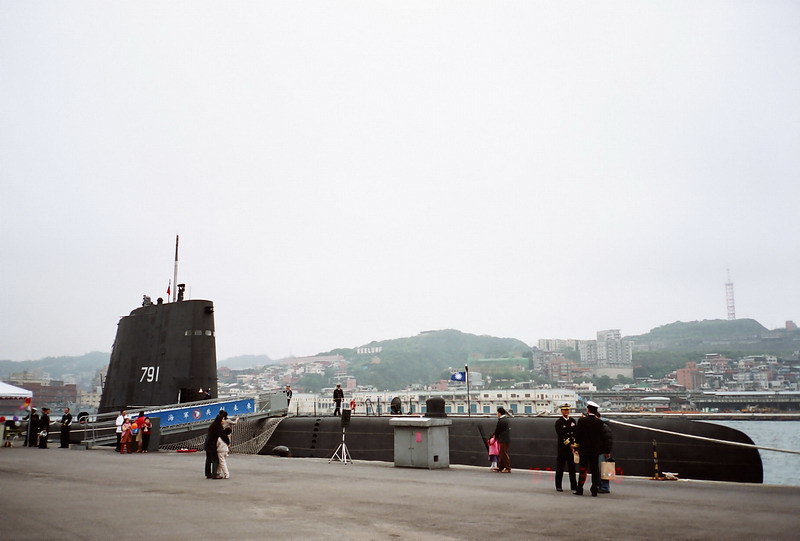The photograph, approximately 6 inches wide and 4 inches tall, captures an outdoor daytime scene featuring a black submarine docked at a harbor. The image is oriented on a concrete platform sloping downward from the left to the right. The submarine, marked with the number 791 in white print, dominates the scene. The distinctive conning tower with white-painted elements and a red-topped post is visible. A metal ramp with a blue banner extends from the submarine to the platform, facilitating access. On the concrete platform, amidst a group of people in dark blue or black uniforms and white hats, a man and woman are seen kissing in the center. To the left, a family of four, possibly of Asian descent, stands near a white tent adorned with colorful balloons. The distant background reveals a cityscape sprawled across a green-clad hillside or mountainside, with indiscernible white lettering on the cliff. The sky above is a dull gray, enhancing the overall somber atmosphere of the scene.